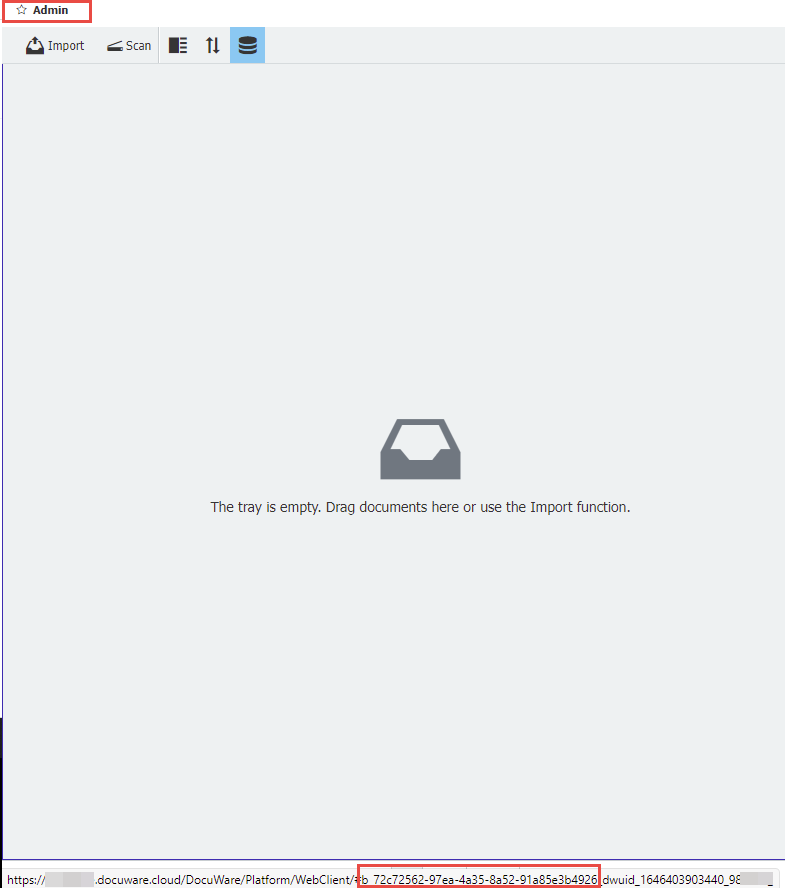The image depicts an administrative upload tool interface with a minimalist design. At the top of the page, there is a rectangular section highlighted in red, featuring the word "Admin" accompanied by a star icon. Below this header, a series of clickable buttons are aligned horizontally. These buttons include: "Import," "Scan," a button with four small notches arranged vertically, another button with an arrow pointing up and an arrow pointing down, and a currently selected button that displays three disks stacked on top of each other.

The main body of the page is largely empty, displaying an icon of an empty folder in the center. Beneath the icon, the text reads: "The tray is empty, drag documents here or use the import function." The entire interface is predominantly light gray, giving a very bare-bones and simplistic aesthetic, with the only other notable color being the white background of the admin section at the top.

At the very bottom, the page's URL is displayed, showing a lengthy web address starting with "https://." Part of this web address is highlighted in a red rectangle for an unspecified reason. Overall, the interface is designed with a clean, uncluttered look, focusing heavily on functionality over visual flair.